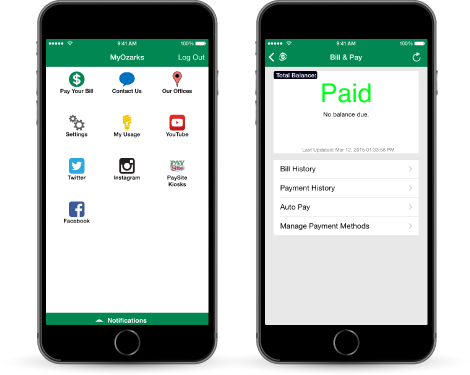This image displays two smartphones side by side, each showing a screen from what appears to be the "My Ozarks" app. 

On the left phone, the screen is labeled "My Ozarks" in a green header with a logout button, indicating that a user is logged in. The main interface includes several options: 
- "Pay Your Bill," represented with a green circle featuring a dollar sign, suggesting easy bill payment functionality. 
- "Contact Us," symbolized by a speech bubble icon, likely for customer inquiries or feedback.
- "Our Offices," directing users to information on office locations.
The second row includes:
- "Settings" for app customization,
- "My Usage" for tracking service usage,
- "YouTube," possibly linking to video resources. 
It also shows icons for "Twitter," "Instagram," and a "Facebook" page, indicating social media connectivity. There is also an option titled "Pay Kiosk."

The right phone screen, still part of the "My Ozarks" app, suggests a transaction completion, displaying "Paid: No Balance Due." This page also has headings for "Bill History," "Payment History," "Auto Pay," and "Manage Payment Methods," offering various financial management options within the app. They appear to have accessed the billing section, after potentially finalizing a payment.